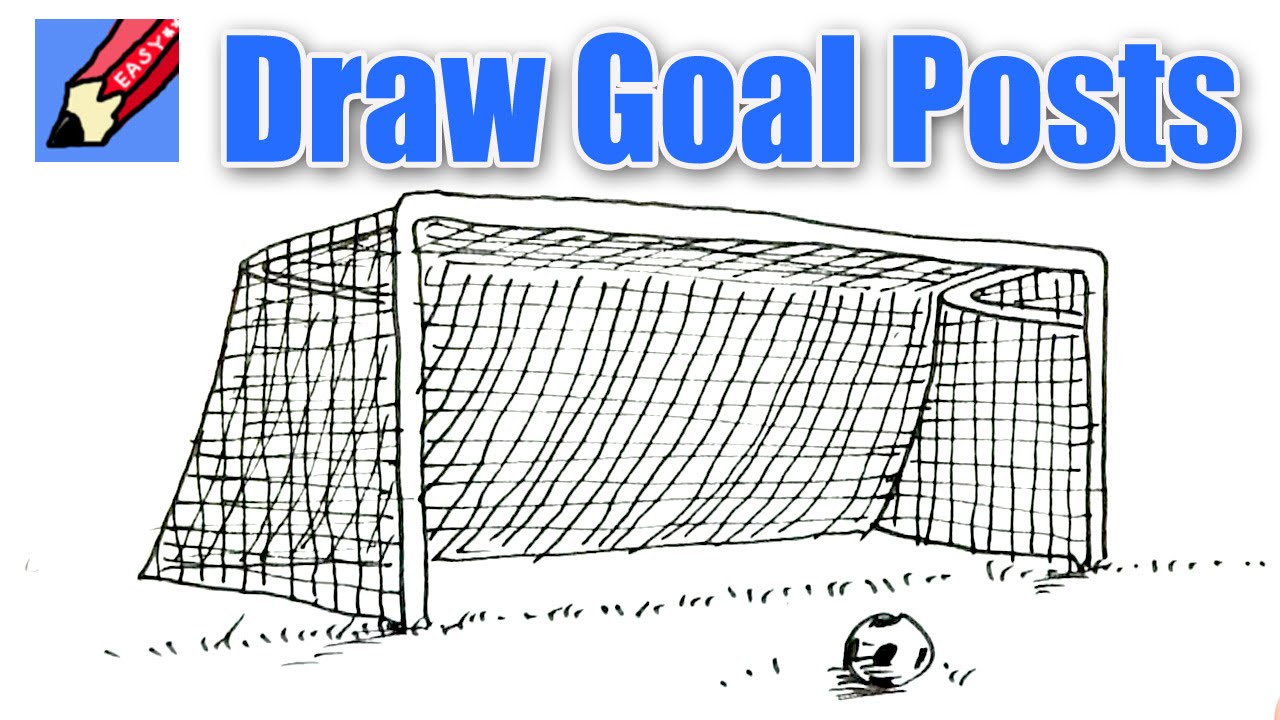The image is an instructional sketch from an art book, designed to teach beginners how to draw a traditional football (soccer) goalpost. At the top of the image, in large blue text with a white border and shadow effect, it reads "Draw Goalposts." To the left of this text, there is a small blue square featuring a red pencil illustration labeled "Easy" in white text. The sketch beneath this header depicts a hand-drawn goalpost, complete with netting and thin lines to suggest grass beneath it. A black-and-white soccer ball is positioned in front of the goalpost. The drawing style is amateur, emphasizing simplicity suitable for novice artists.